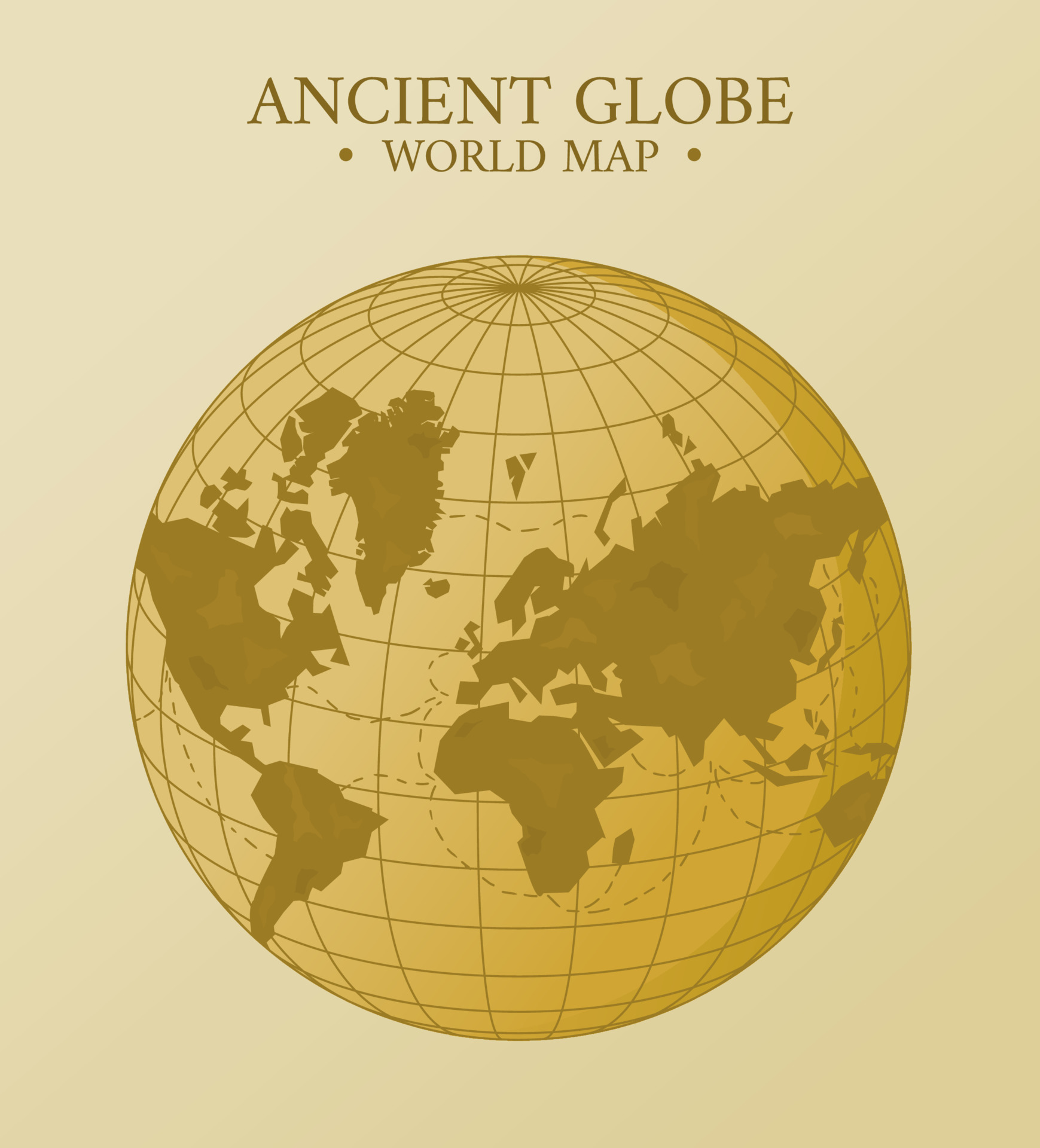The image features a detailed colored sketch or lithograph rendered in varying shades of brown and gold on a tan background. At the center of the composition is a large globe, where the continents of North America, South America, Asia, Africa, and a small segment of Australia are depicted in silhouette. The ocean areas are filled in with a light tan color, contrasting with the darker tones of the continents. The globe is marked with both longitudinal and latitudinal lines, as well as some cross-hatching to indicate additional geographical details. Above the globe, in capital letters and brownish print, it reads "ANCIENT GLOBE," with "WORLD MAP" separated by two bullet points below it. The design suggests an antique or historical aesthetic, with no additional foreground text, reinforcing its classic and simplified portrayal of the world’s geography.